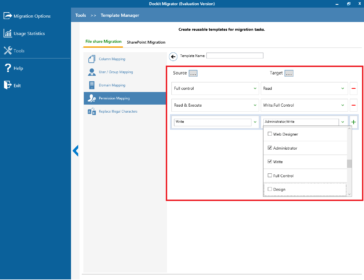This image captures a slightly blurry webpage, with the content just discernible. On the left side and across the top of the page, a dark blue background features white text, creating a clear navigational or header section. Below this, a lighter blue section with white writing sits prominently. Centered beneath these blue sections, a white box stands out against the background. Just below the lighter blue bar, black text introduces two selectable options.

The first option, displayed in green font, has a yellow bar directly underneath it. The alternative choice is written in black font, positioned adjacently. The green font selection appears to be active, indicating user choice, and the fourth option in a subsequent list is also selected. At the bottom of the image, the chosen option is highlighted by a red box, requiring the user to input specific information to proceed. This detailed arrangement suggests a form or survey interface with clear indicators for user interaction.